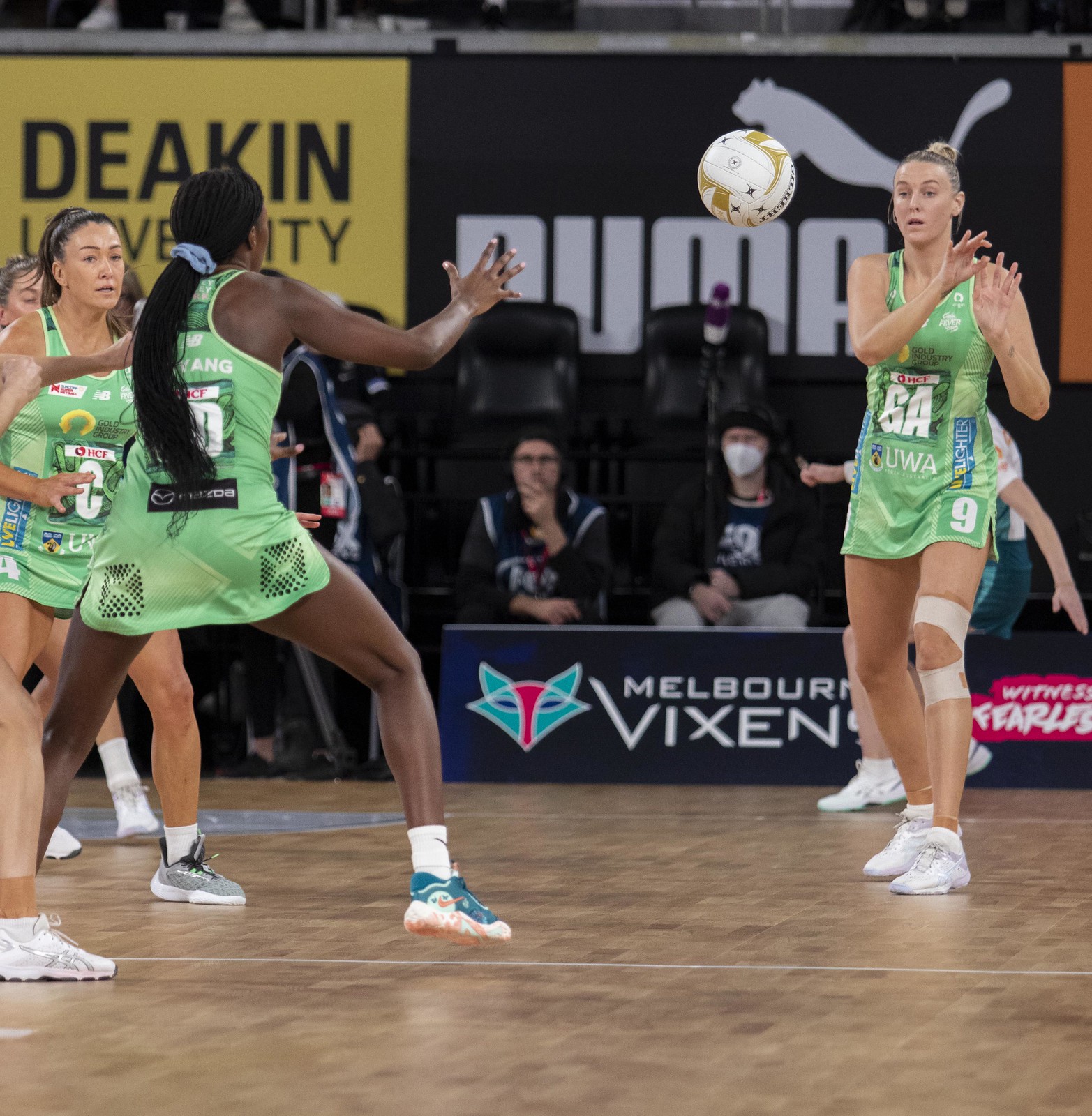In a vertical rectangular action shot from a women’s basketball game, the scene unfolds on a traditional wooden court. The focal point is three players in matching green tank top jerseys with printed numbers, depicting a cohesive team effort. One player, a Caucasian woman with her hair tied back in a bun, stands to the far right with a surprised expression on her face, likely having just passed a white and gold ball to her teammate. This teammate, a black woman with a long ponytail reaching down her back, has her hands up, ready to receive the pass. To the black woman’s left, another Caucasian teammate watches intently, poised with her hand down. Behind the players, three men sit on a bench in front of a wall adorned with signage, including 'Melbourne Vixens,' 'Deakin,' and a large Puma logo. The dynamic moment is capped by details like the players' revealing one-piece uniforms that expose their thighs, amplifying the intensity and athleticism of the game.